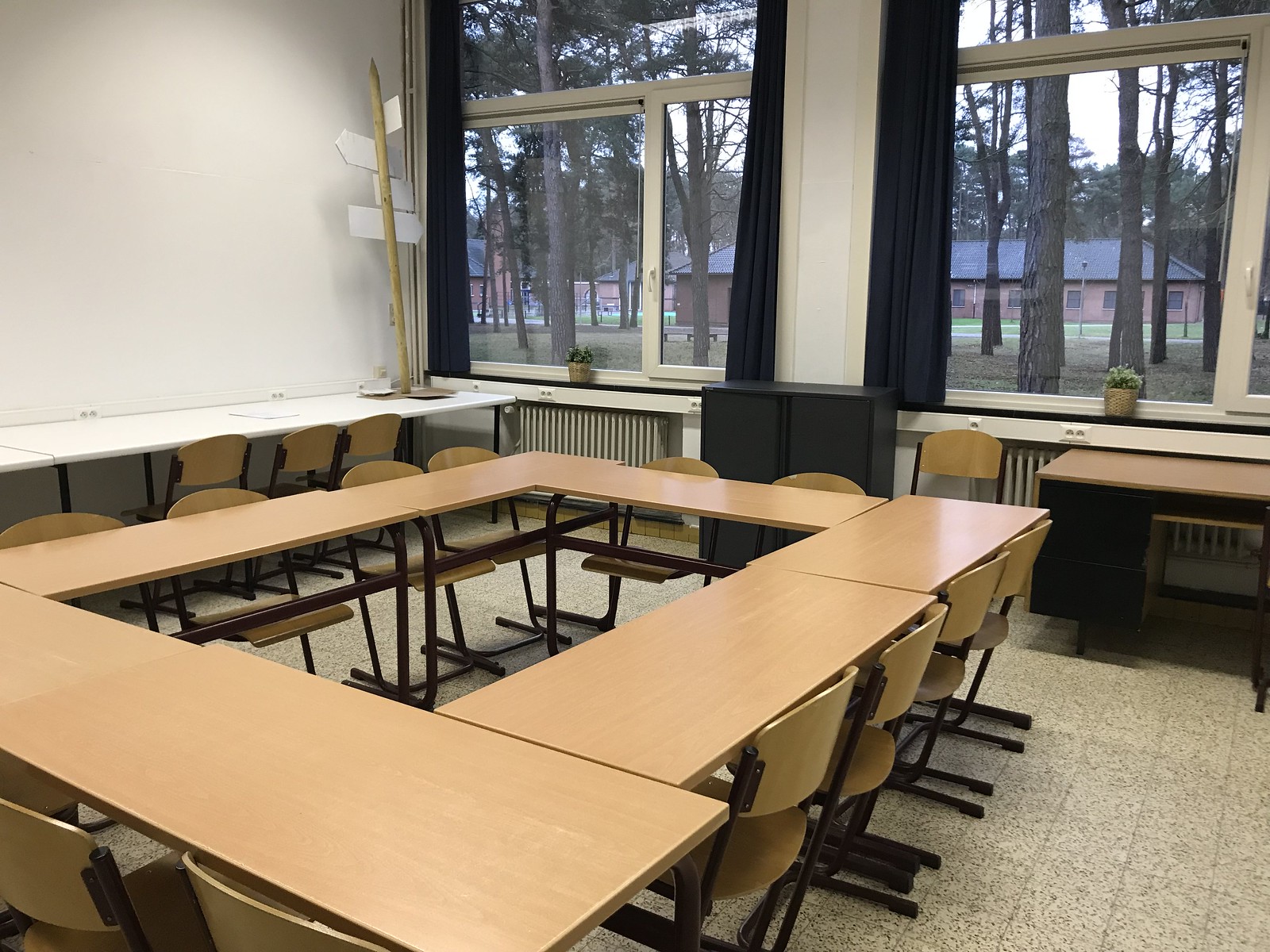The photo depicts a room featuring a series of light wood, rectangular desks, configured into a larger rectangle with an open rectangular space in the middle. There are seven such desks, each accompanied by two chairs situated across from each other. These chairs have a tan wooden backrest and a cushioned seat, supported by black or brown metal frames. The floor is covered in gray tiles with numerous black speckles, resembling granite, each tile being a small square.

In the background, on the left side of the image, a large, clear window with white borders is visible. Through this window, tall trees with brown trunks and green leaves can be seen, as well as distant buildings characterized by black pyramid-like roofs and brown or red walls. To the left of the rectangular desk arrangement, some white tables with additional chairs are noticeable. Also in the background on the left, a pole with directional arrows sits atop one of the tables, contributing to the room's functional setup.